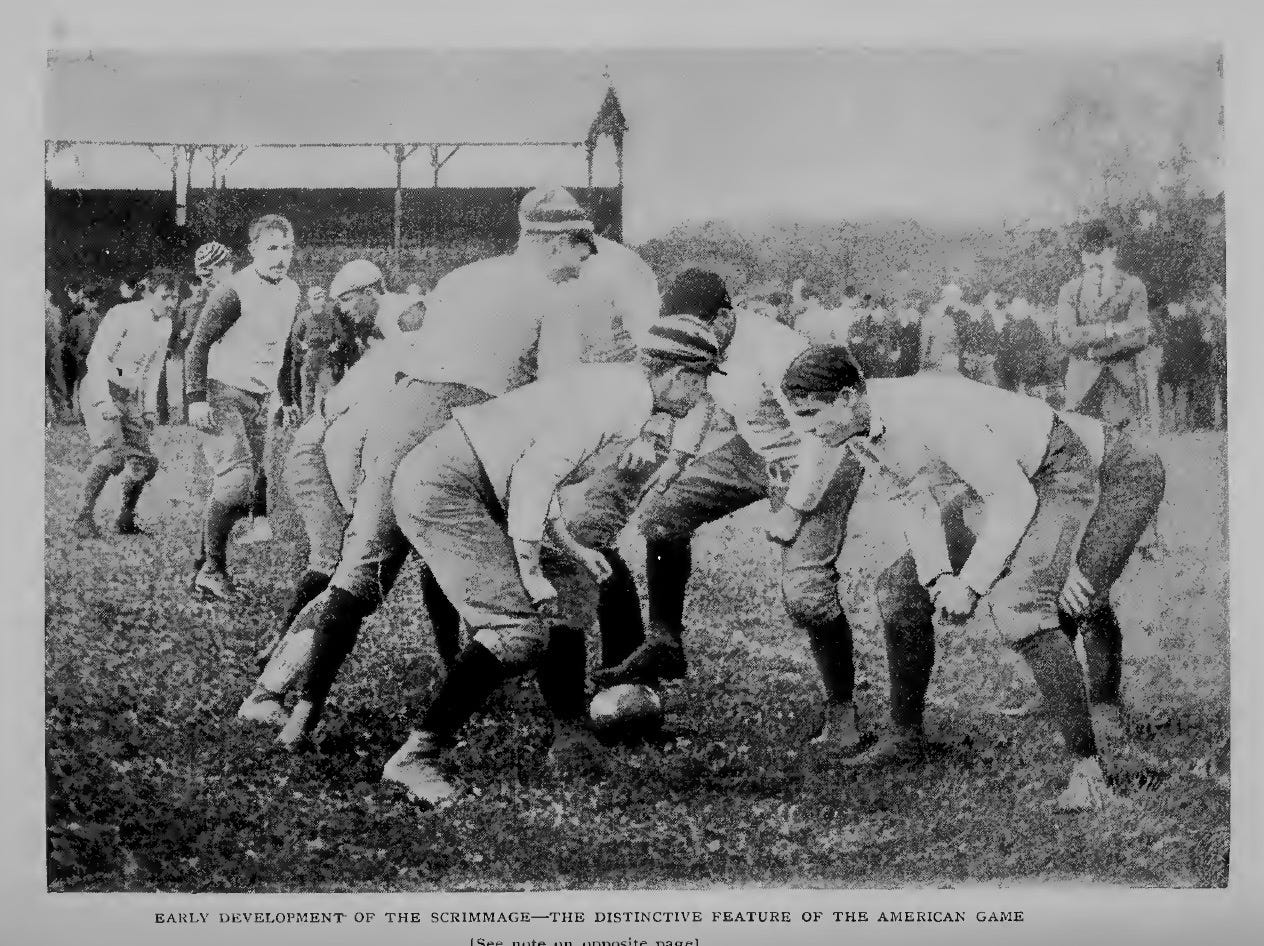This historical photograph captures a scene from the early development of American football, dating likely from the early 1900s to the 1920s. The image showcases a group of men or boys engaged in a scrimmage, a foundational element of the game as indicated by the caption, "early development of the scrimmage, the distinctive feature of the American game." The players are dressed in period-appropriate attire, including white shirts, knee-length shorts paired with high socks, and shoes. Some players also don knit caps. One player prominently positions his foot on the ball, suggesting an imminent play. In the background, muted grandstands and a cluster of spectators add context to the setting. A coach, distinguishable by his sport coat, shirt, tie, and top hat, observes from the right side of the frame. The photograph, rendered in black and white, exudes a sense of nostalgia, offering a glimpse into the nascent stages of American football.